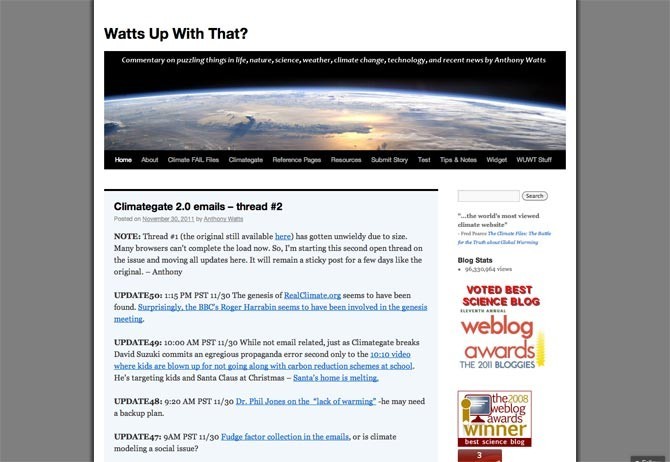The image captures a blog page with a clean, white background and black text, prominently featuring the title "Watts Up With That" stylized with "WATTS" referencing electrical wattage. At the top of the page, an image shows the curvature of the Earth, suggesting a focus on global issues.

Directly below the title, a navigation menu provides several options: "Home," "Climate Fail Files," "Climategate," "Something Pings," "Resources," "Sub Slicy Test," "Wildcat WLNC Stuff." The main content showcases a blog post titled "Climategate 2.0 Emails - Thread Number Two," which includes numerous updates and discussions. Users are reminded that the first thread is still available for use.

On the right-hand side, a sidebar runs from the middle of the page down to a search bar at the bottom. The sidebar displays blog statistics, spotlighting over 96 million views, and boasts accolades such as "Voted Best Science Blog by Weblog Awards" and "2008 Weblog Awards Winner."